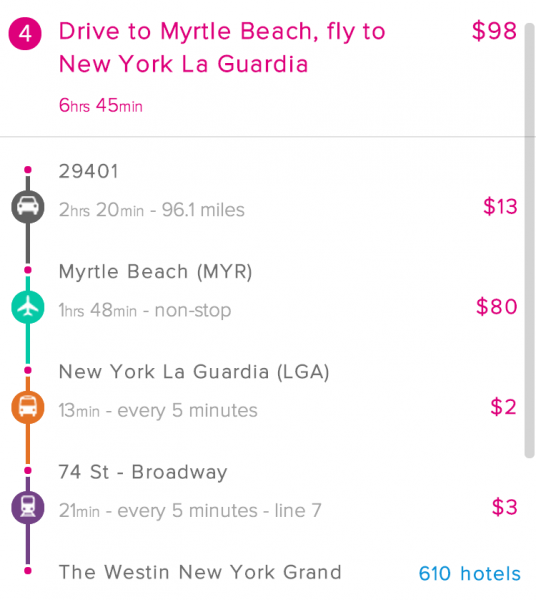Image Caption:

At the top left of the image, a hot pink circle with a white numeral "4" sits prominently. Adjacent to the circle on the right, text in hot pink reads, "Drive to Myrtle Beach, fly to New York, LaGuardia." Further to the right, there is a hot pink dollar sign followed by the number "98." Below this line, in smaller hot pink font, the text "6 hours 45 minutes" appears, where "HRS" and "MIN" are significantly smaller than the numbers "6" and "45" respectively. A light gray divider beneath this section effectively separates it from the timeline of the person's travels.

The timeline begins at the top with the text "29401" in gray. Directly below, in a lighter shade of gray, it reads "2HRS 20MIN - 96.1 miles." To the right of this information, a hot pink dollar sign is followed by the number "13," indicating a cost of $13. To the left, a car icon is displayed against a gray circle.

Descending further into the timeline, we enter a green section featuring a plane icon within a green circle that has a slight teal tint. This segment is labeled "Myrtle Beach (MYR)" in gray. Underneath, in lighter gray and smaller font, it indicates a duration of "1HRS 48MIN - non-stop." Further right in hot pink, the cost is marked as "$80."

Following this part, the background shifts to orange, displaying a circular icon with a white bus inside. Next to this icon, the text "New York LaGuardia (LGA)" is found in gray. Below this, in lighter gray and smaller font, it notes "13MIN - every 5 minutes," where "every 5 minutes" is slightly larger than "13MIN." To the right, the price in hot pink reads "$2."